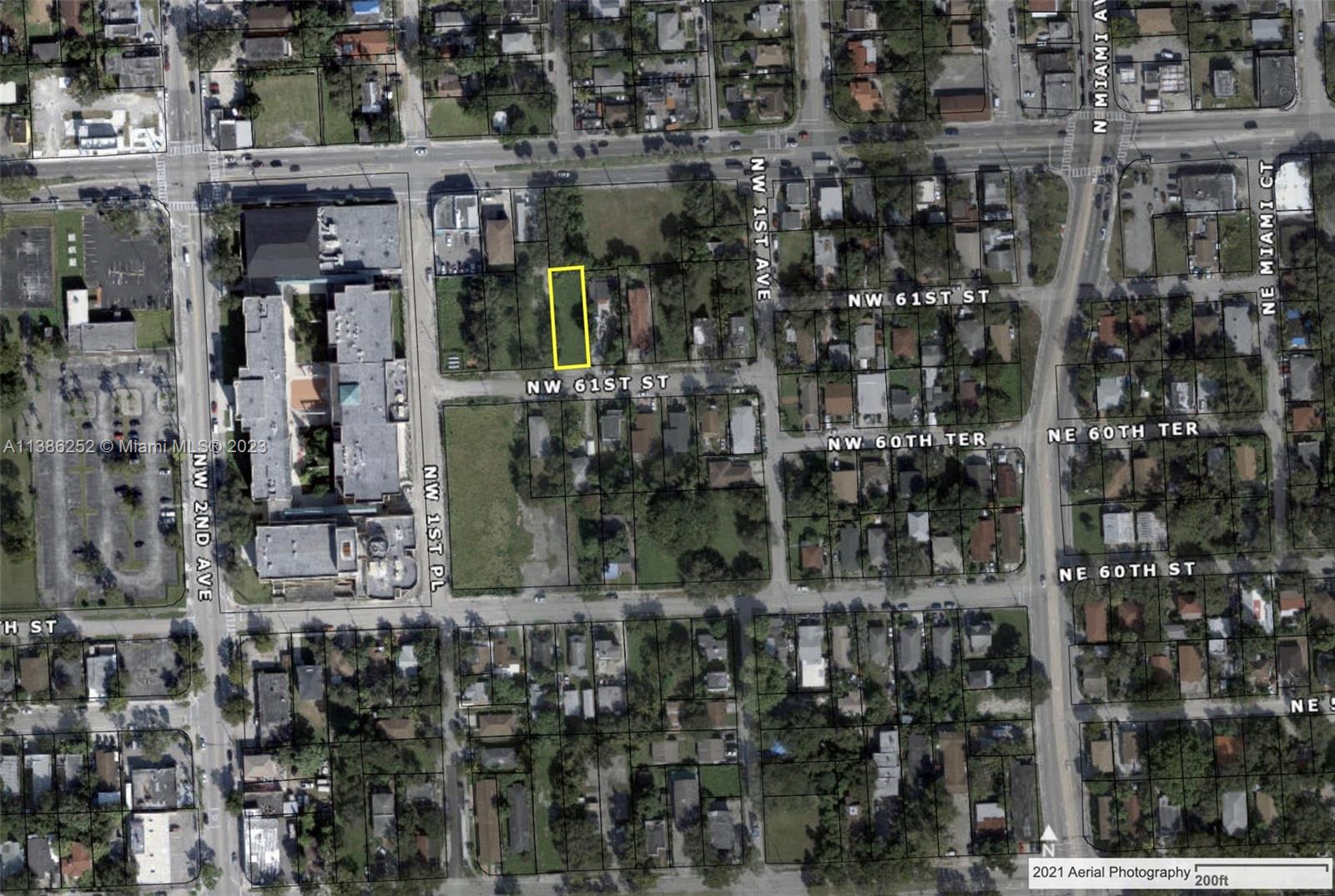This aerial mapping image, taken from a satellite, showcases a suburban neighborhood with a prominent focus on a rectangular plot of land highlighted in yellow. This plot is centrally located between Northwest 1st Place and Northwest 1st Avenue, near Northwest 61st Street. The map features superimposed road names, providing a clear grid layout of the area. Horizontally, the roads include Northwest 61st and Northwest 60th Streets, while vertically, notable streets include Northwest 2nd Avenue, a wide thoroughfare, and Northwest 1st Avenue. The image captures a mix of residential areas with houses of various colors, predominantly gray, brown, and red rooftops, amidst a lush green background indicating abundant tree coverage. Scattered throughout the neighborhood are larger, more rectangular buildings suggestive of small office buildings or strip malls, indicating some commercial presence. The streets don't follow a strict grid pattern, adding to the unique layout of this vibrant community.